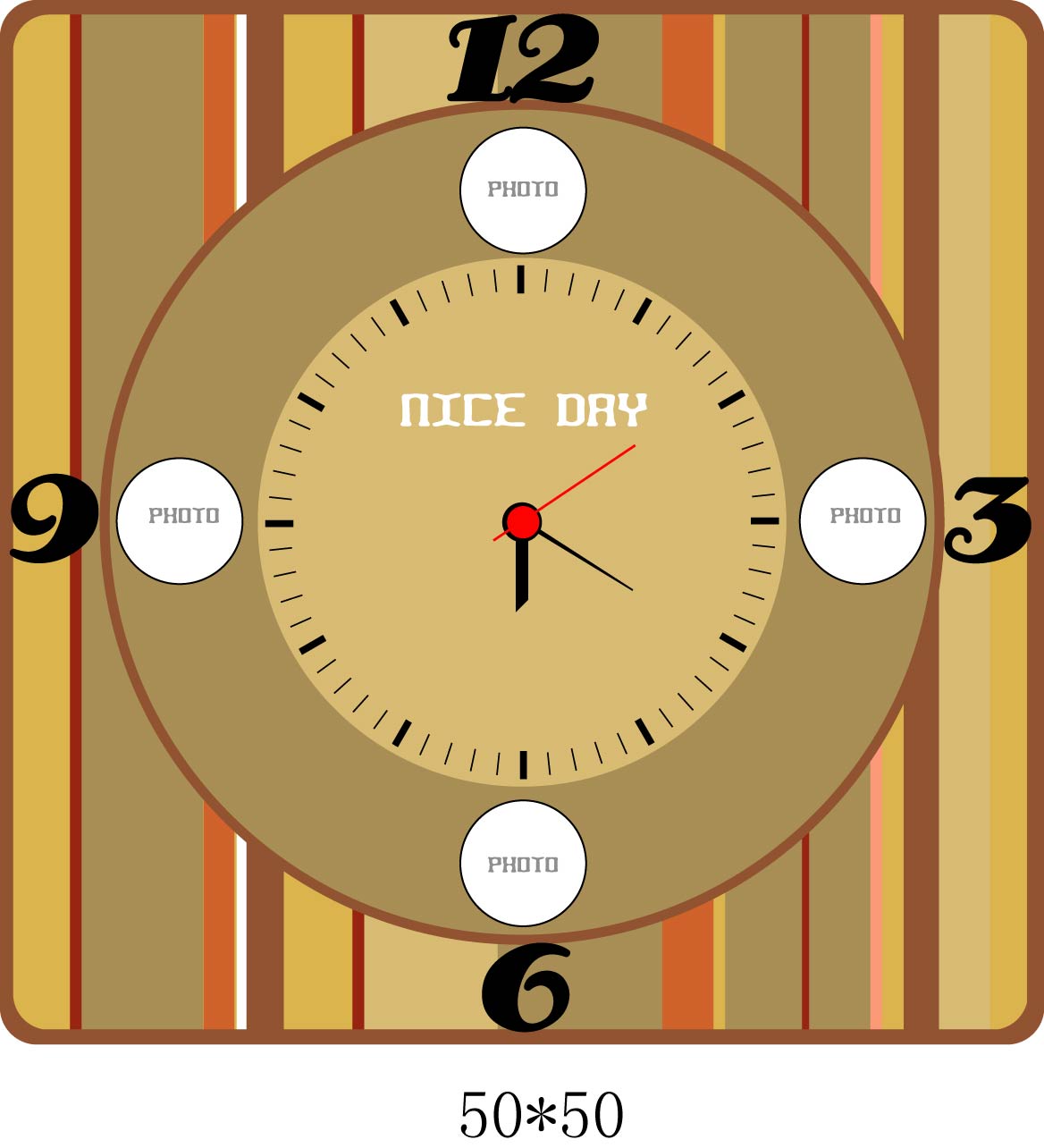This image is a detailed poster drawing of a retro-style clock, reminiscent of the 1970s. The clock is centrally placed within a large square frame outlined in an intensive brown. This frame is filled with vertical stripes of varying widths in a palette of beige, gray, burnt orange, white, dark brown, gold, peach, red, and pink, creating a vibrant, multi-colored background.

The clock face itself features large black numbers at the 12, 3, 6, and 9 positions, and adjacent to each of these numbers is a black-outlined circle labeled "photo" in white text, suggesting spaces for photographs. The center of the clock face is light beige, marked with the phrase "nice day" in white lettering. The clock hands, showing the time as approximately 6:20, are black for the hour and minute hands and red for the second hand. Below the clock face, there is an inscription reading "50 times 50."